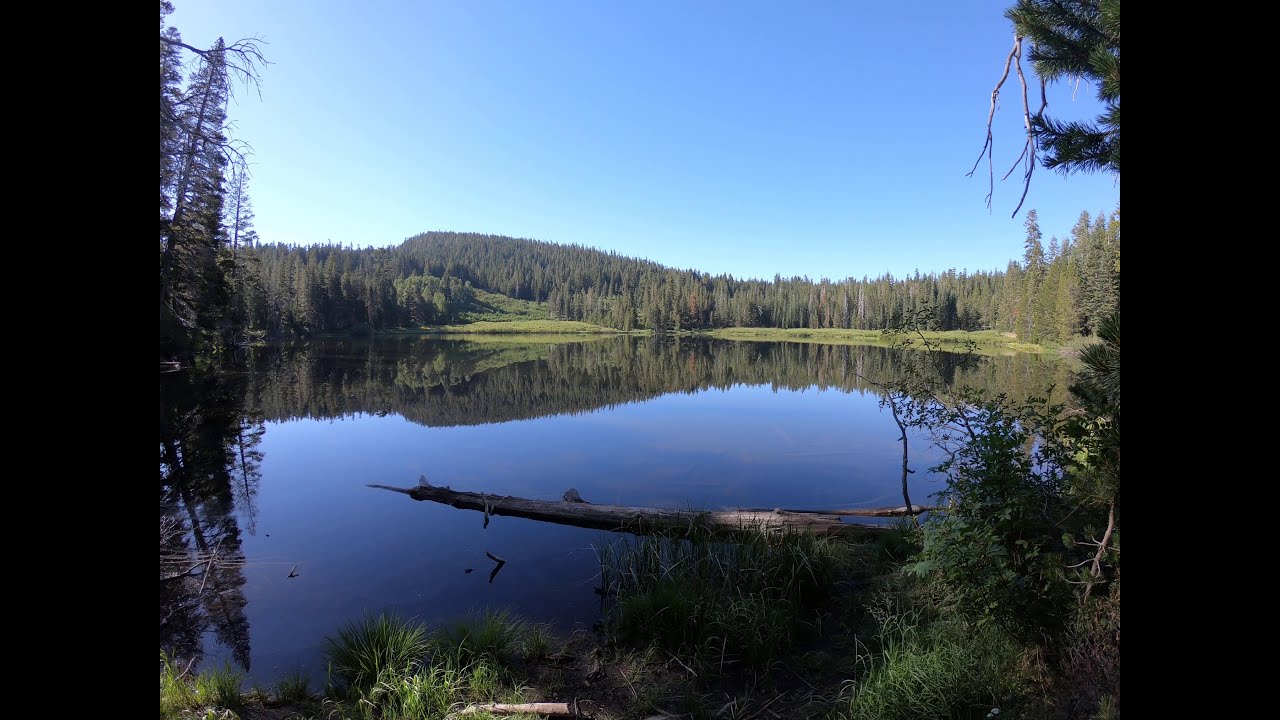This is a highly detailed, color landscape photograph capturing a serene, glassy lake that dominates most of the scene. The clear, blue, daytime sky beautifully reflects off the still water, creating a seamless blend of green and blue hues. The lake is surrounded by a picturesque environment featuring a mix of tall, dark green pine trees and slightly frosted areas behind the lake, indicative of a cold climate.

On the far shoreline, a slight hill is densely covered with various trees and grass. The left side of the image has a vertical black stripe, adding a contrasting element to the composition. More trees and branches are visible on both the left and right edges, further enhancing the natural ambiance.

In the foreground, where the viewer stands on a grassy section of land, lies a prominent fallen log partially submerged in the water, slightly off-center towards the right. The immediate shoreline is dotted with additional shrubs, grass, and weeds.

The overall scene is so tranquil and idyllic, with perfect reflections and rich colors, that it resembles a painting and stands as a testament to photographic realism.